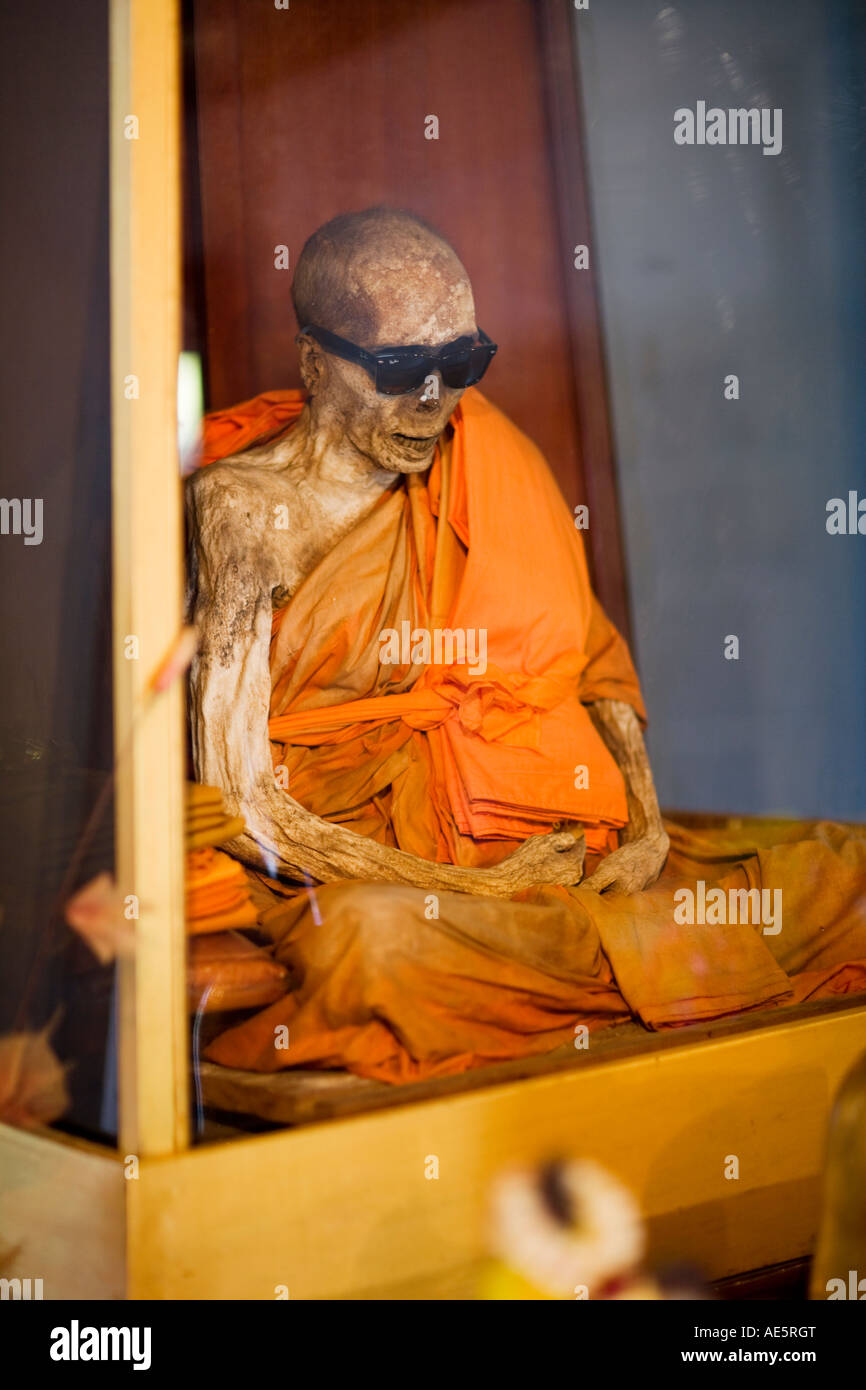This color photo depicts a mummified Buddhist monk sitting in a traditional cross-legged meditation pose. His skeletal arms rest in his lap, with his hands positioned at the center of his legs. The visible parts of his body include his right shoulder, the lower portion of his left arm, and his withered, bald head. His mouth is open, clearly showing his teeth, and he dons an unexpected pair of black sunglasses. Despite his mummified state, he wears the vibrant orange robes characteristic of Buddhist monks. The monk is encased in a display case framed in teak wood. Watermarked text, featuring lowercase 'a' letters and the name "Alamy," is scattered across the photograph. A black band at the bottom left corner includes the Alamy logo, an image ID number, and the website www.alamy.com.